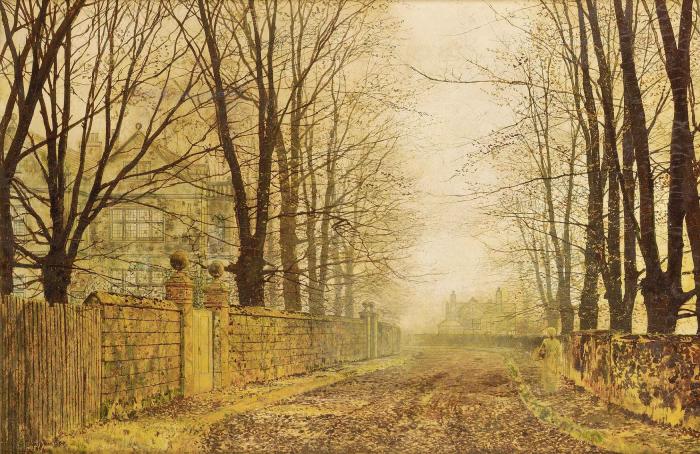This hand-painted image captures a serene outdoor scene reminiscent of the English countryside, featuring a collection of manor houses and fall foliage rendered in muted autumnal colors of browns, golds, and yellows. On the left side of the image, there is a large house, partly concealed by trees that have shed most of their leaves. A quaint dirt road runs through the middle, flanked by varying types of fences; on the left side, it transitions from an old wooden fence to stone, highlighted by two sets of stanchions topped with round balls, indicating gated entrances. The right-hand side of the road is bordered by a stone wall made of small stones, resembling an old-world sidewalk. In the far background, another expansive manor house is visible, adding depth and suggesting considerable estates. The scene captures a tranquil moment in nature, with no people or animals visible, allowing the viewer to fully appreciate the picturesque and detailed autumn landscape.